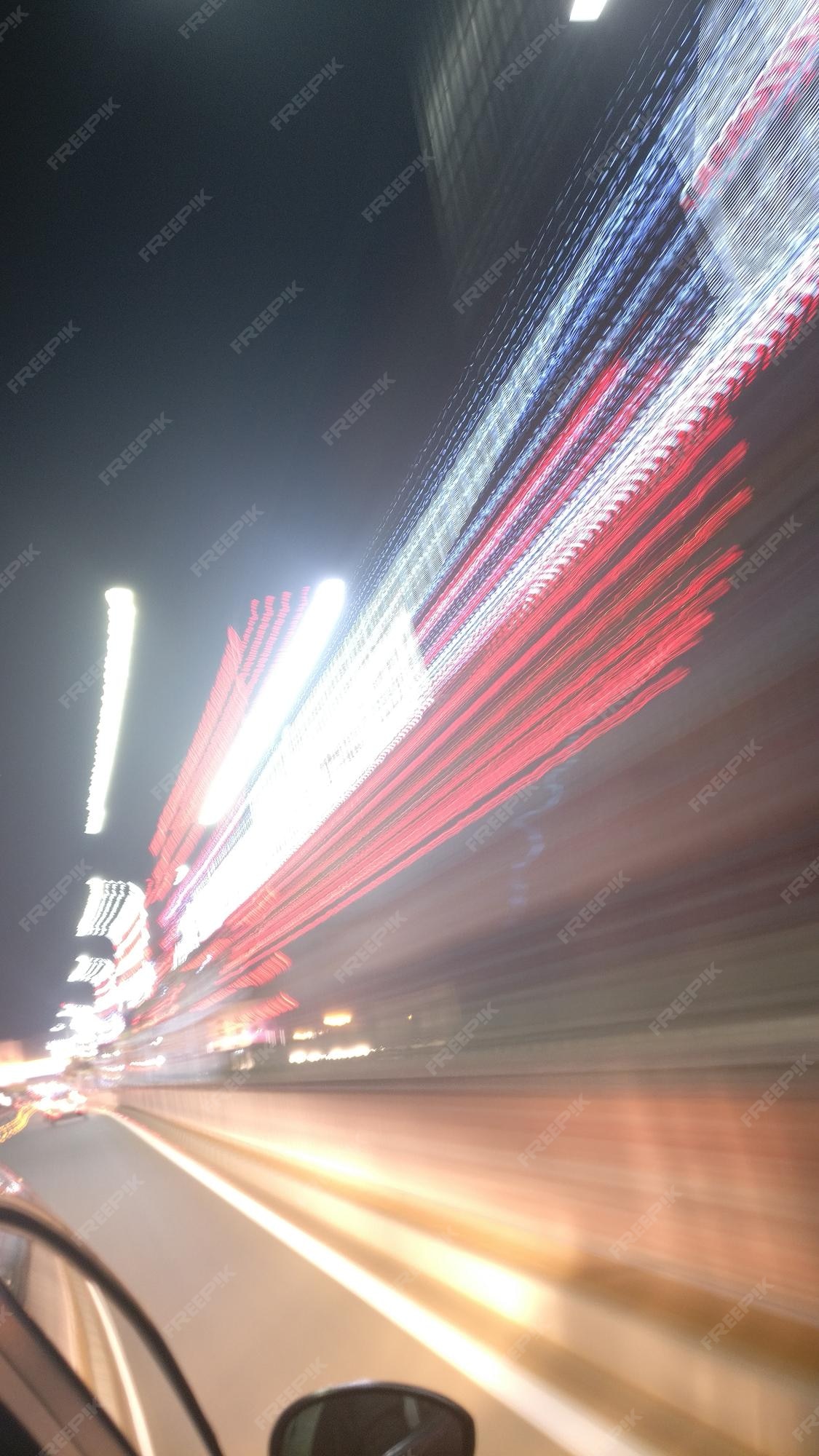The image captures the dynamic motion of a car driving down a highway, photographed from the perspective of someone inside the vehicle. The scene is dominated by blurred lines of red, white, and tan, indicative of the car's speed. The lower left corner reveals partial views of the car's side window and rear-view mirror, emphasizing the perspective from inside the vehicle. The road is just visible in this corner, while the rest of the image is a vivid display of streaked lights, creating an almost NASCAR-like effect. In the distance, another car is faintly visible, also blurred by motion. A repetitive watermark reading "Freepik," with the 'I' upside down, is superimposed over the entire image, indicating its source.